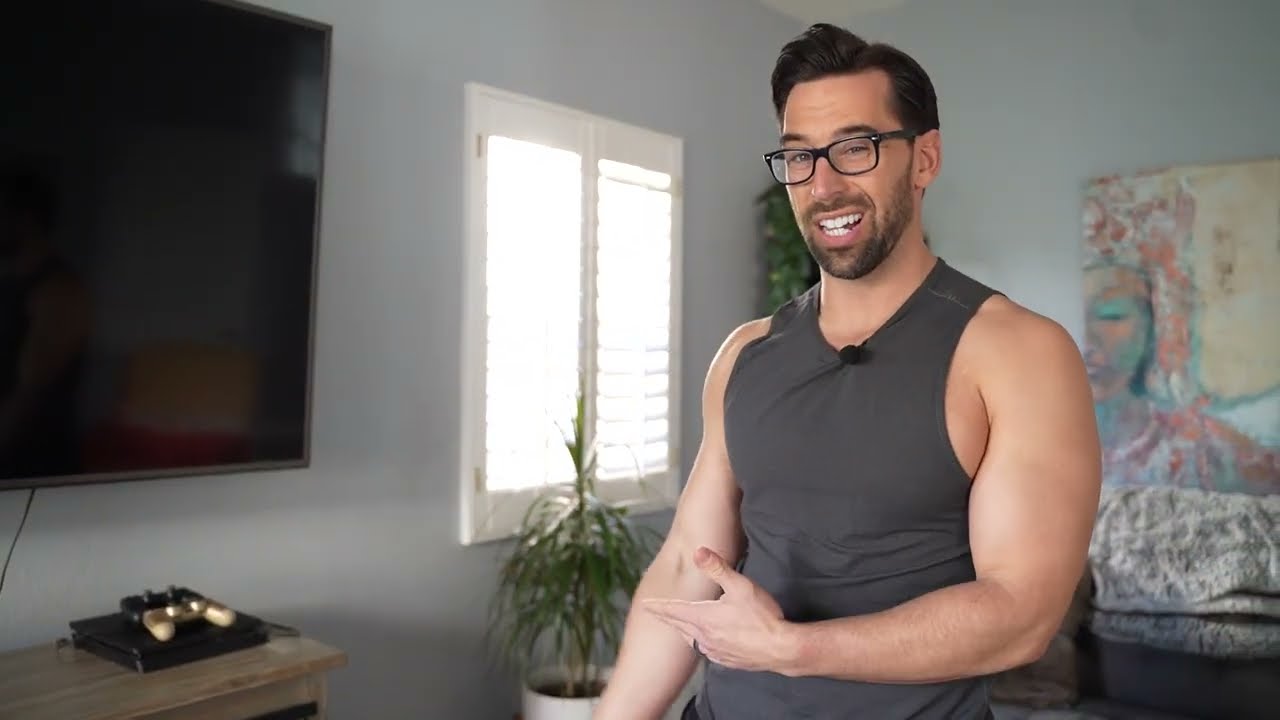In this detailed screen grab of what appears to be a YouTube or social media video, we see a well-lit room, likely lit by a ring light, which captures a muscular man in his late 30s mid-conversation. He sports a gray muscle shirt, black glasses, and a well-groomed beard and mustache. His hair, styled with mousse, is slicked to the right. He has a small microphone around his neck, indicating he is capturing audio for the video. 

The man, with a slight smirk on his face, gestures towards a large TV on the wall to his right, below which sits a PlayStation 4 console with a black and a white controller on top. A gold-colored device, possibly another controller, is also visible on the table beneath the TV. Behind him, a pastel-colored painting and a small green Dressena Marganata houseplant sit beneath a window. The background includes a couch with a blanket over it, and the room features gray and white walls intersecting at a 90-degree angle. The setting suggests this might be a video tutorial, review, or commentary filmed in a living room or a bedroom.